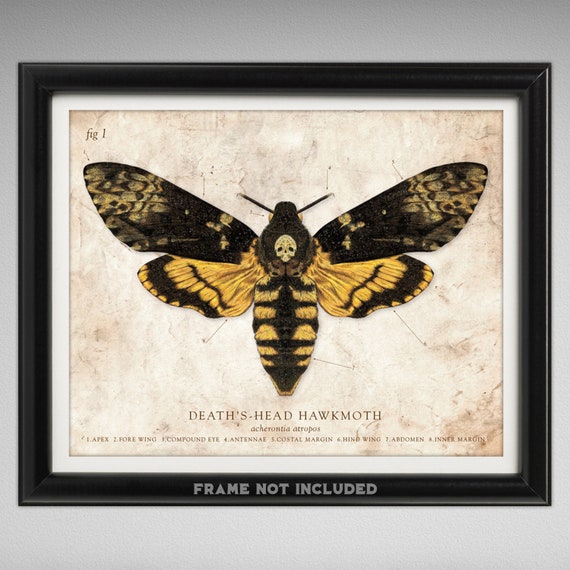This image depicts a detailed, framed illustration of a Death's Head Hawk Moth, labeled as "Agromedia Atropis." The drawing is positioned in a black frame and set against a gray wall. The illustration is created on paper that mimics the appearance of old, oxidized, and faded script paper, enhancing the vintage aesthetic.

The moth, displayed in a top-down view, features striking colors: the two larger forewings are primarily black with hints of yellow near the edges, while the smaller hindwings are predominantly yellow accented by black tips. Its abdomen is distinctly striped in black and yellow. Notably, a white skull is intricately drawn on the main body near the head, which is a characteristic marking of this species. The moth also has yellow eyes and two black antennae.

Accompanying the illustration, there is text underneath identifying the moth and providing labels for various anatomical parts: "1 apex, 2 forewing, 3 compound eye, 4 antenna, 5 coastal margin, 6 hind wing, 7 abdomen, 8 inner margin." Below this educational labeling, the frame itself has a message stating "frame not included" in white silhouette, adding a contemporary note to the otherwise classic presentation.